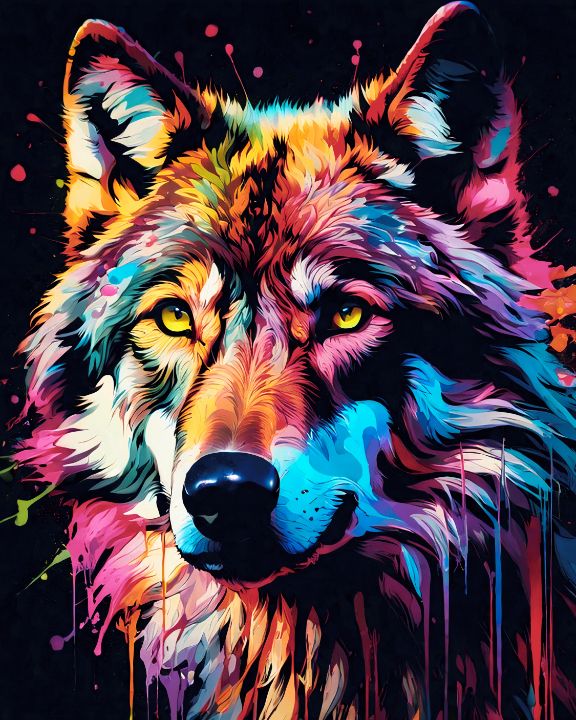This surreal digital painting features a vividly colored wolf set against a black background, accented with paint splotches. Dominating most of the image, the wolf's fur melds into a rainbow of bright pink, orange, yellow, blue, white, and green hues. Its stylized, almost paint-like texture creates an illusion of the fur melting off its body. The wolf's rounded ears stand tall, and its large, reflective black button nose contrasts sharply with its white and pink-highlighted muzzle. The wolf, seen from the chest up, turns slightly to the left, as if looking at something over the viewer's shoulder, with expressive yellow eyes and a bemused, almost smiling expression. The paint seems to drip from various points on the wolf, adding to the whimsical, artistic feel of the piece. The background, though predominantly black, features intentional paint splatters of blue and pink, further enhancing the surreal, dreamlike quality of the artwork.